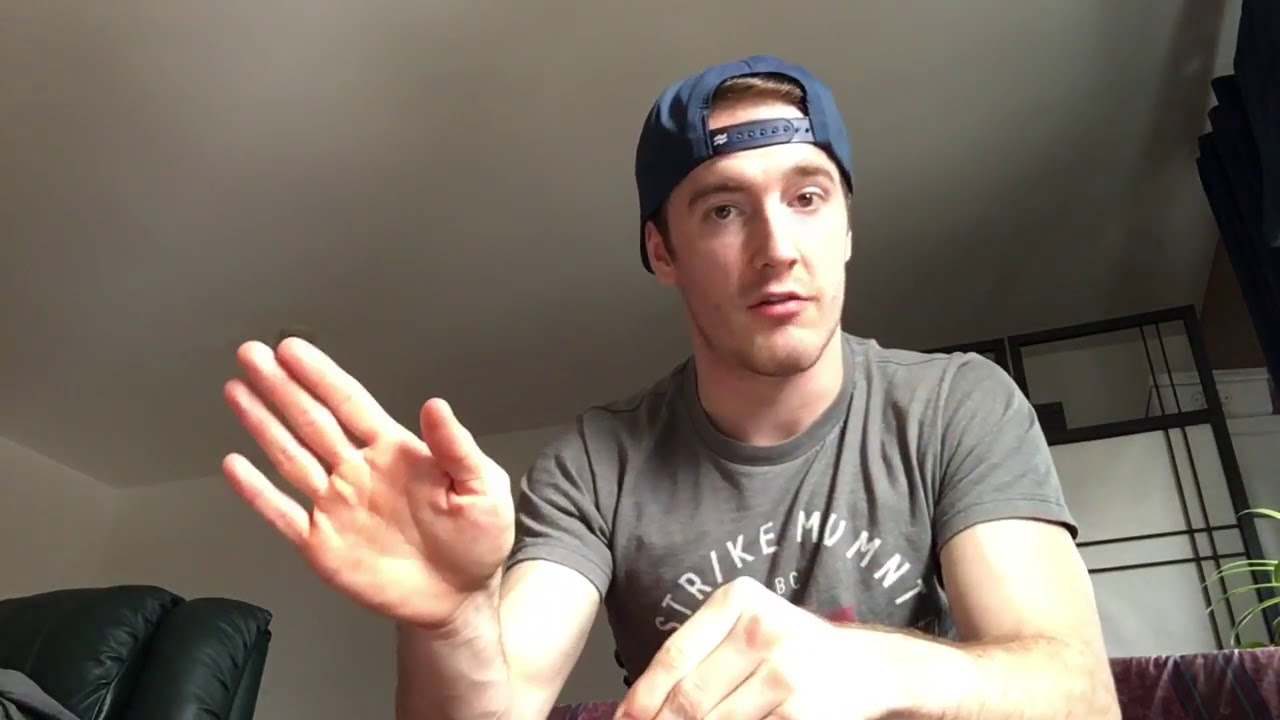This image depicts a young Caucasian man with brown hair and brown eyes, likely in his 20s, seated and waving into the camera. He is in a room with white walls, which appears to be a living room. He is wearing a gray short-sleeved t-shirt with white text that reads "Strike M-U-M-N-T B-C." The man has a slight stubble, indicating he hasn't shaved for a couple of days, and he is sporting a backwards navy blue trucker cap. One of his arms is resting flat against a surface, probably a desk, while the other arm is bent at the elbow, with his hand raised in a waving gesture. Behind him, there is a black-framed picture and a partially visible green plant. To his left, there is a gray leather chair and, behind him, a cabinet with a clear door and a leather chair with a purple cover draped over it.